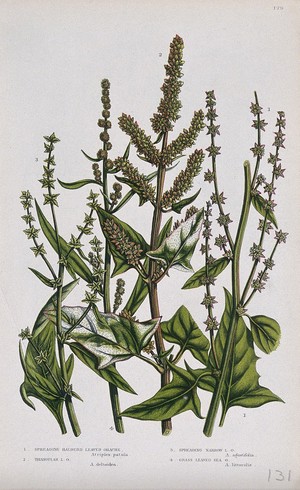This detailed illustration shows a cluster of plants on what appears to be a small postcard with a plain white background, labeled "131" at the bottom right corner. The primary focus is on four distinct branches, three of which are green and one brown. The green branches exhibit vibrant, star-shaped leaves with three pointy ends - two on the sides and one at the top. These mature leaves feature some sort of white covering. The various plants on the postcard vary in structure; some display spiky, tightly-grouped green buds while others have smaller leaves and sprout delicate white flowers or seed pods from their stems. The brown branch in the center is unique, showcasing clusters of seed-like buds instead of flowers. Overall, the illustration emphasizes a mix of green foliage and brownish flowers against a white backdrop, creating a vivid contrast. At the very bottom, there is some nearly illegible text, possibly labeling the four different types of plants depicted.